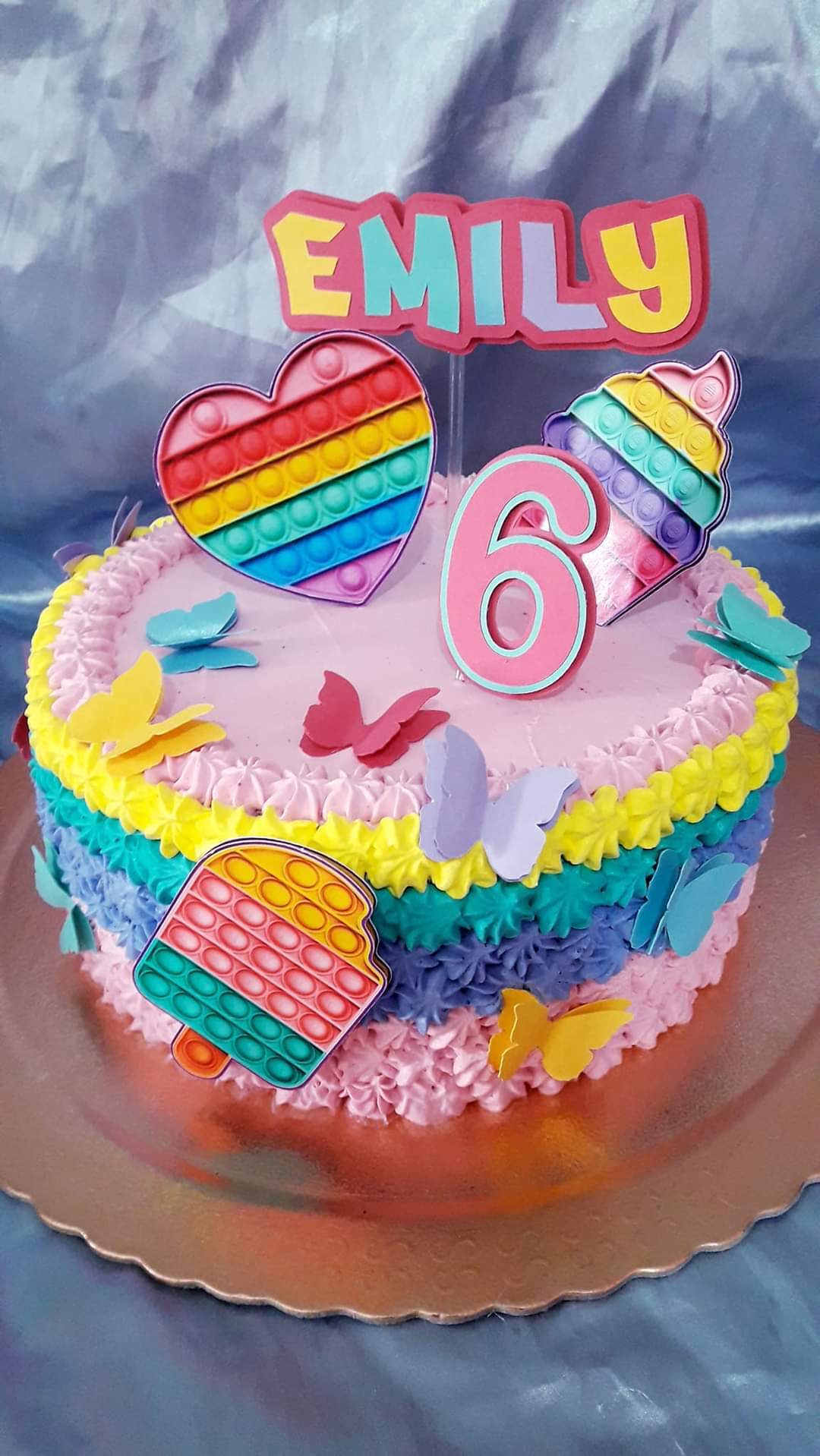This photograph captures an elaborate, colorful birthday cake designed for Emily’s sixth birthday. The cake, placed prominently in the center of the image, is mounted on a silver scalloped-edged platter and set against an iridescent purple fabric backdrop, which also forms the base underneath it. The cake features multiple vibrant layers, alternating in lavender, yellow, and dark purple shades, all intricately piped with icing. Adorned with an array of decorative elements, the cake showcases a mix of whimsical paper butterflies in colors such as blue, yellow, red, green, and lavender, complementing the cake's layered hues.

Additionally, the cake is topped with three small butterflies matching the cake’s palette, along with several colorful fondant or toy decorations, including a rainbow-colored ice cream cone, heart, and cupcake. A large pink number six stands atop the cake, alongside Emily's name, which is displayed on a small sign attached to a toothpick. The edges and top of the cake are decorated with stars in varying colors, including lavender, yellow, teal, purple, and pink, adding to its festive appearance. To complete the setup, the cake is presented on a brass and silk serving tray, enhancing the overall celebratory ambiance of the scene.